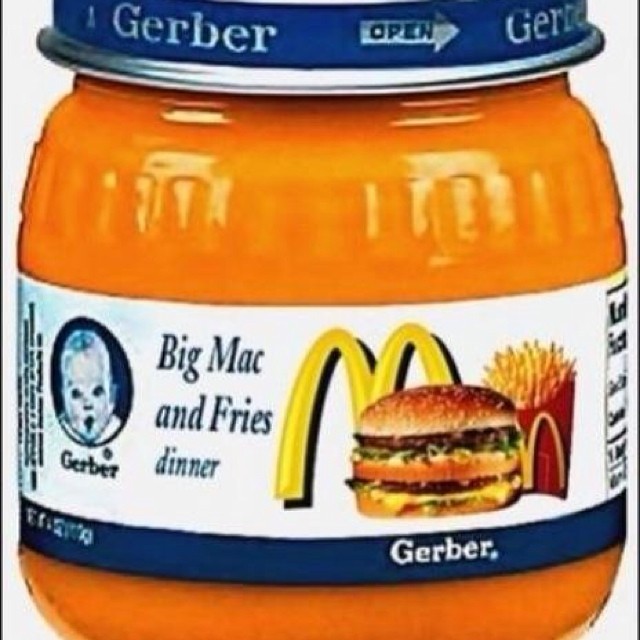A detailed photograph showcases a Gerber baby food jar prominently. The jar features a dark blue cap adorned with the silver text "Gerber" and an arrow indicating the direction to turn for opening. This satirical product is humorously branded as "Big Mac and Fries Dinner" flavored baby food, complete with a neon orange hue that mimics a bright neon shade. The label amusingly includes the iconic McDonald's logo alongside a tempting image of a large hamburger and fries, enhancing the parody. Additionally, the label displays the classic Gerber baby logo in dark blue with a white baby face, repeated alongside the Gerber brand name at the bottom. The whimsical nature of the product suggests it's an attention-grabbing and playful concept, likely not available as an actual baby food flavor.